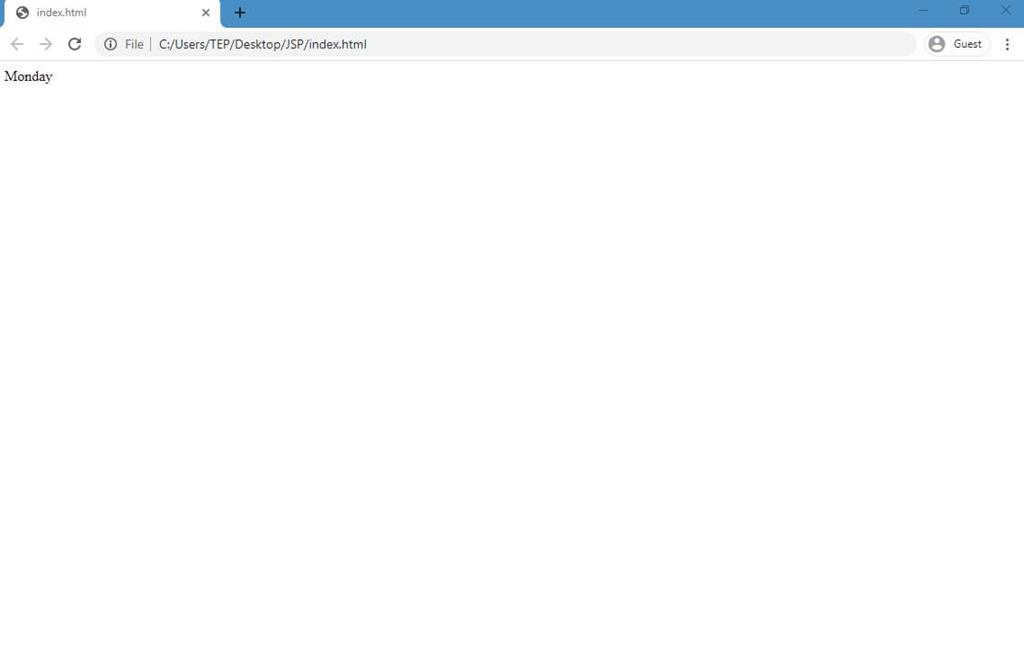The image depicts a basic web browser interface with a single open tab. The open tab presents a minimalistic design, with the only visible text being "Monday" at the top. The tab itself is labeled in all lowercase as "index.html" and is accompanied by a globe icon. To the right of the tab label, there's a standard "X" button to close the tab. Adjacent to this, a blue bar with a "+" symbol allows for the addition of new tabs. On the far right of the toolbar, options to minimize, switch, or exit the browser are present, indicated by a minus symbol, a tab-switching icon, and a close icon, respectively.

Below this main toolbar, there are navigation arrows for moving back and forth between pages, a refresh button, and a file path displayed as "C:/user/TP/Desktop/JSP/index.html". To the right, it indicates the browser is being used by a guest, denoted by "Guest" with three trailing dots.

Underneath the address bar, the page content displays simply a large capital "M" representing Monday. The overall appearance is stark and minimal, with no additional information or imagery present.